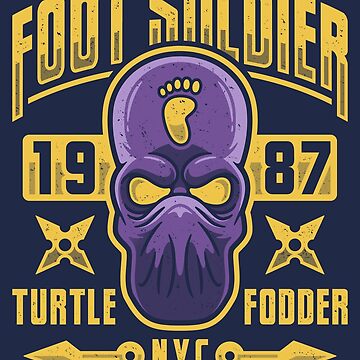The image is a detailed graphic with a prominent focus on an unusual, alien-like face. The face is purple with oval-shaped, yellow eyes and a nose, but no visible mouth. Strikingly, there is a yellow footprint imprinted on the creature's forehead. Surrounding this central face, there is text in bold yellow. The words "FOOT SOLDIER" are placed above the head, while "1987" is split on either side of the face, creating a balanced design. Below this, there are two golden-yellow ninja stars flanking the words "TURTLE" and "FODDER," contributing to a martial arts theme. At the very bottom of the image, "NYC" is inscribed. The text "1987" is uniquely highlighted with blue against a yellow backdrop, while the entire image is framed within a darker blue background, making the yellow text stand out vividly.